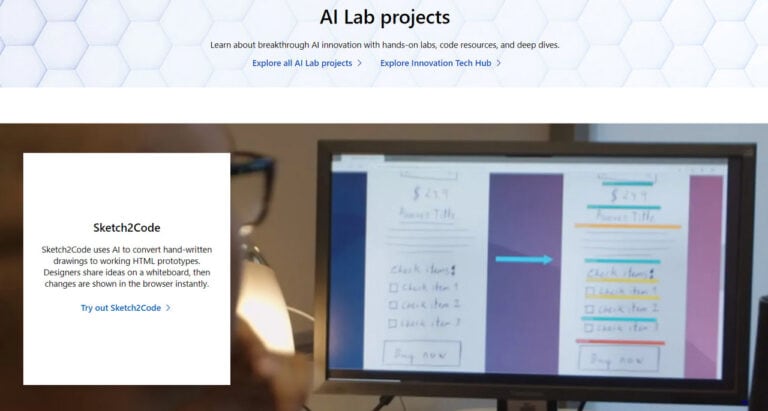This image showcases a design page displayed on a laptop or monitor. To the left of the screen, text reads, "Sketch to Code," highlighting an AI-powered tool designed to transform Android 10 sketches into functional HTML prototypes. It emphasizes the seamless process where changes are immediately reflected in the browser. At the top, the section titled "AI Labs" invites users to delve into pioneering AI advancements, offering hands-on labs, coding resources, and in-depth explorations. A call to action encourages viewers to explore all AI Lab projects and innovations from the comfort of their homes.